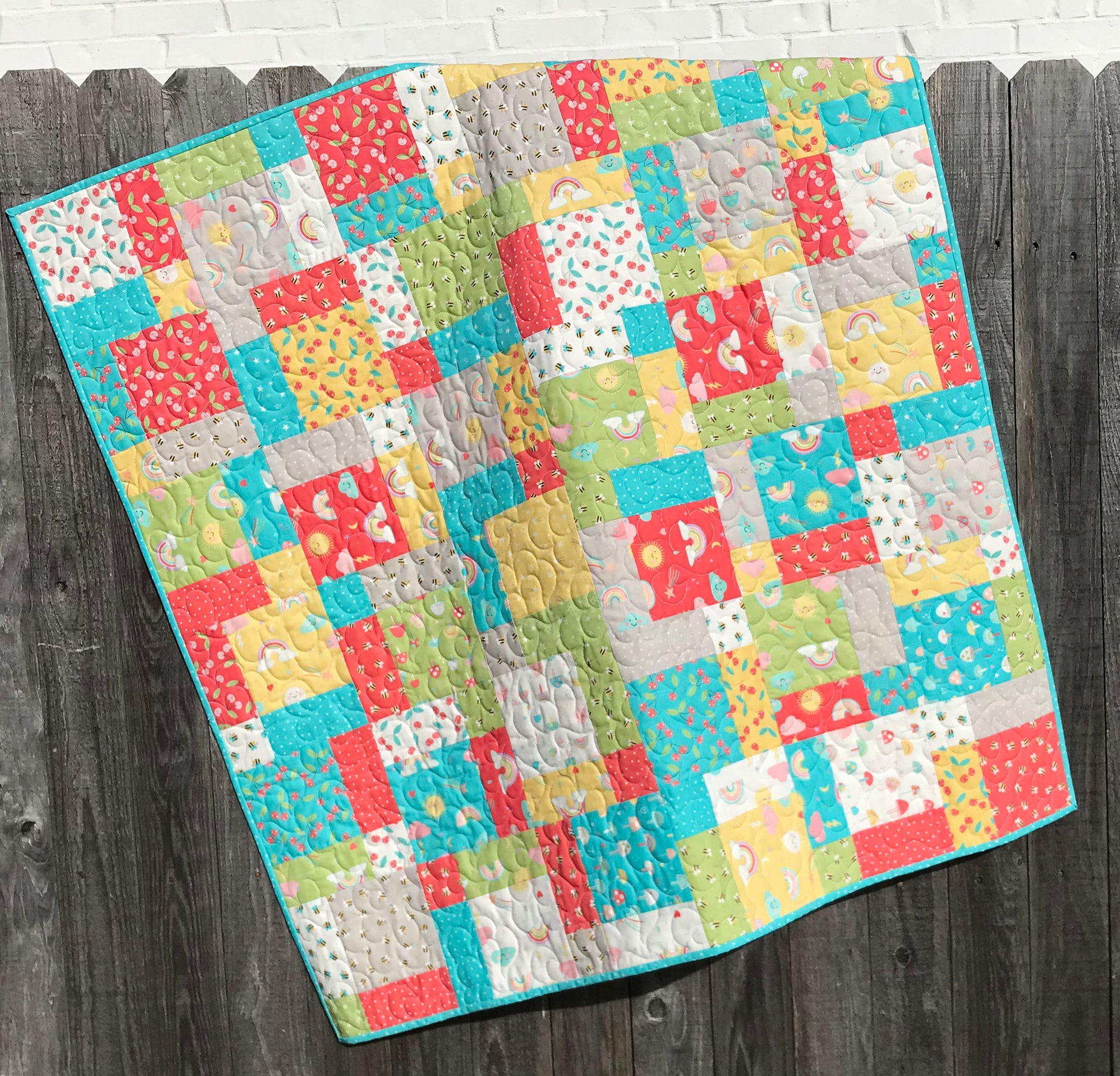The image depicts a wooden fence with uniform slats that are weathered to a grayish-brown hue. Draped over the top of this fence is a vibrant, patchwork quilt that appears to be designed for a baby or child. The quilt features an eclectic array of patterns and colors, including shades of light blue, yellow, red, white, green, and a bubblegum pink. Each patch or shape on the quilt is adorned with playful, kid-friendly motifs such as cherries, strawberries, rainbows, smiling suns, smiling clouds, bumblebees, mushrooms, and various fruits. The quilt is meticulously crafted using a combination of squares and rectangles, with some sections highlighting curved quilted patterns. The overall design is both cheerful and whimsical, perfectly complementing the rustic texture of the weathered wooden fence.